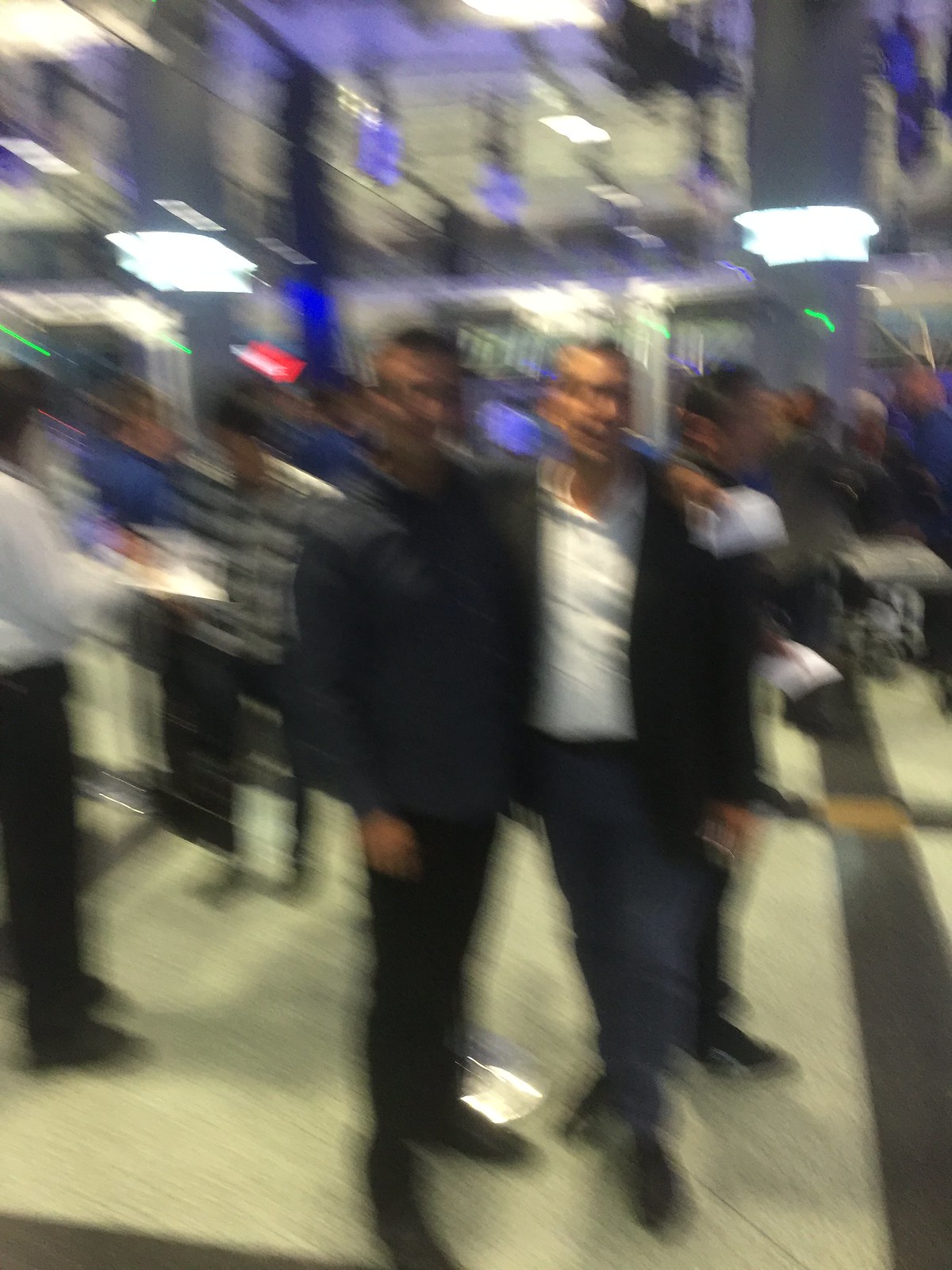In an out-of-focus photograph, two men stand side by side, their arms around each other, in a bustling lobby that appears to belong to a hotel or a similar communal space. The man on the left is dressed entirely in black, wearing a long-sleeved jacket, a shirt underneath, pants, and shoes of the same color. He stands adjacent to a metal stanchion, often used to hold velvet ropes, which is partially visible with its base near his left foot. He faces the camera directly.

His companion to the right sports a dark jacket over a white collared shirt, notably missing a tie, along with blue jeans and dark shoes. They are surrounded by at least six other individuals, who are scattered throughout the background, adding to the lively atmosphere of the scene. 

The lobby features a reflective ceiling, and possibly a similarly reflective wall on the left side of the image. In the background, on the right, a pillar adorned with a light fixture at its top casts reflections on both the wall and ceiling, contributing to the overall ambiance of the space.